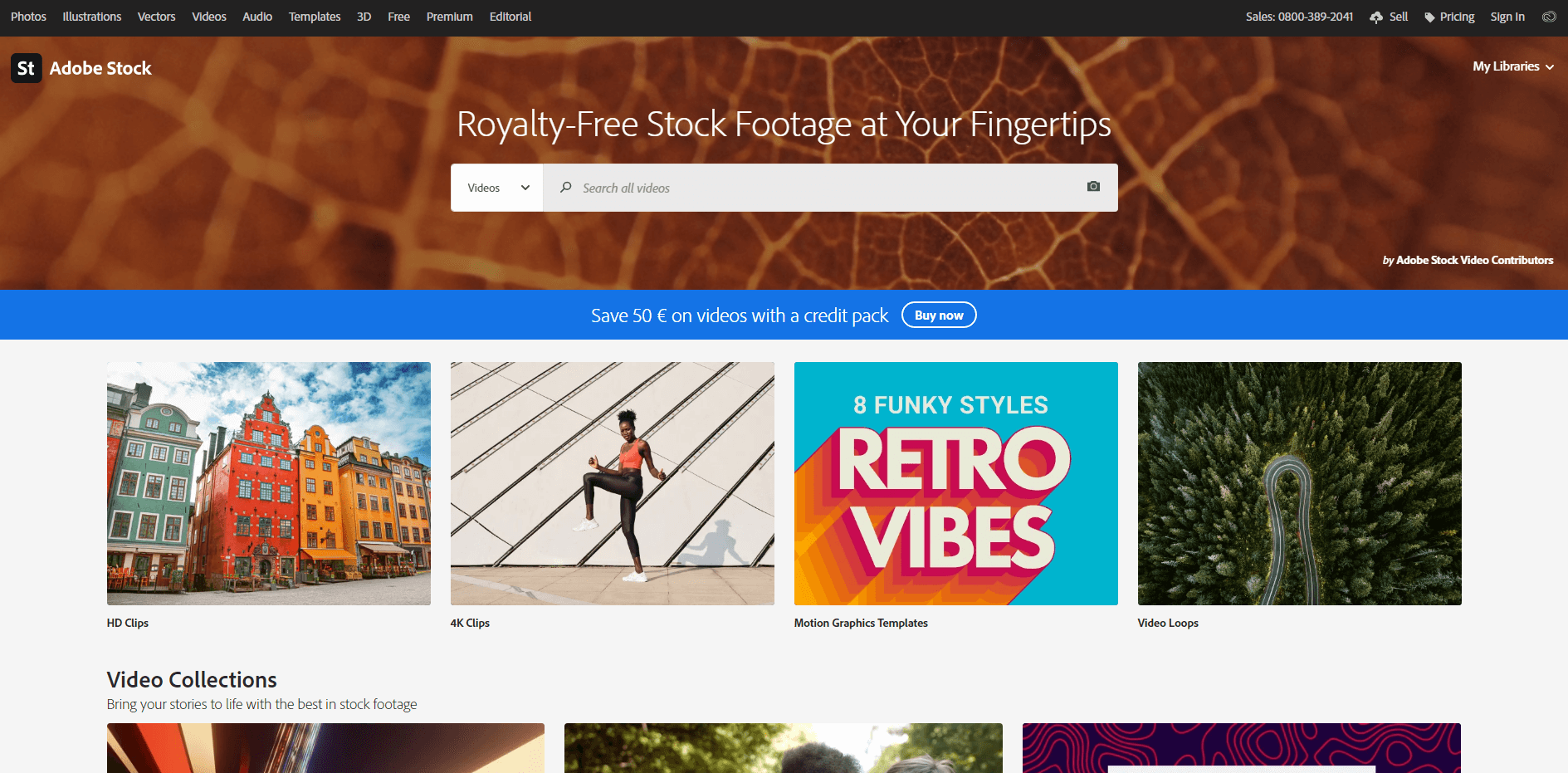At the top of the image is a rectangular section featuring giraffe-like patterns in dark and light orange hues. In the top right corner of this rectangle, "Adobe Stock" is written in white letters. Centered within the rectangle, also in white lettering, is the text "Royalty-Free Stock Footage at Your Fingertips." Below this are two white rectangles, a smaller one atop a larger one, with the larger rectangle containing a search button that partially says "Search All," though the complete text is obscured.

Beneath these rectangles is a blue rectangle bearing the message "Save 50% on Video with Credit Pack. Buy More." Further down are four evenly spaced squares. The first square showcases an image of buildings or houses in various colors—one aqua, one orange, and three yellow. The second square features a photograph of a black woman jump-roping. She is dressed in an orange tank top and black pants, with white tennis shoes, one leg in the air and the other slightly bent. Her shadow is visible against a white, glass-like wall, and she is standing on a cement floor.

The third square has text that reads "Eight Funky Styles Retro Vibes." The fourth square contains an indistinct image showing an object protruding from the ground, as viewed from above, with a shape resembling a jelly bean in the center.

Below these squares, three more squares are partially visible, capped by the text "Video Collection. Bring your stories to life with the best in stock footage." The images within these squares are not fully visible, making it difficult to identify their contents.